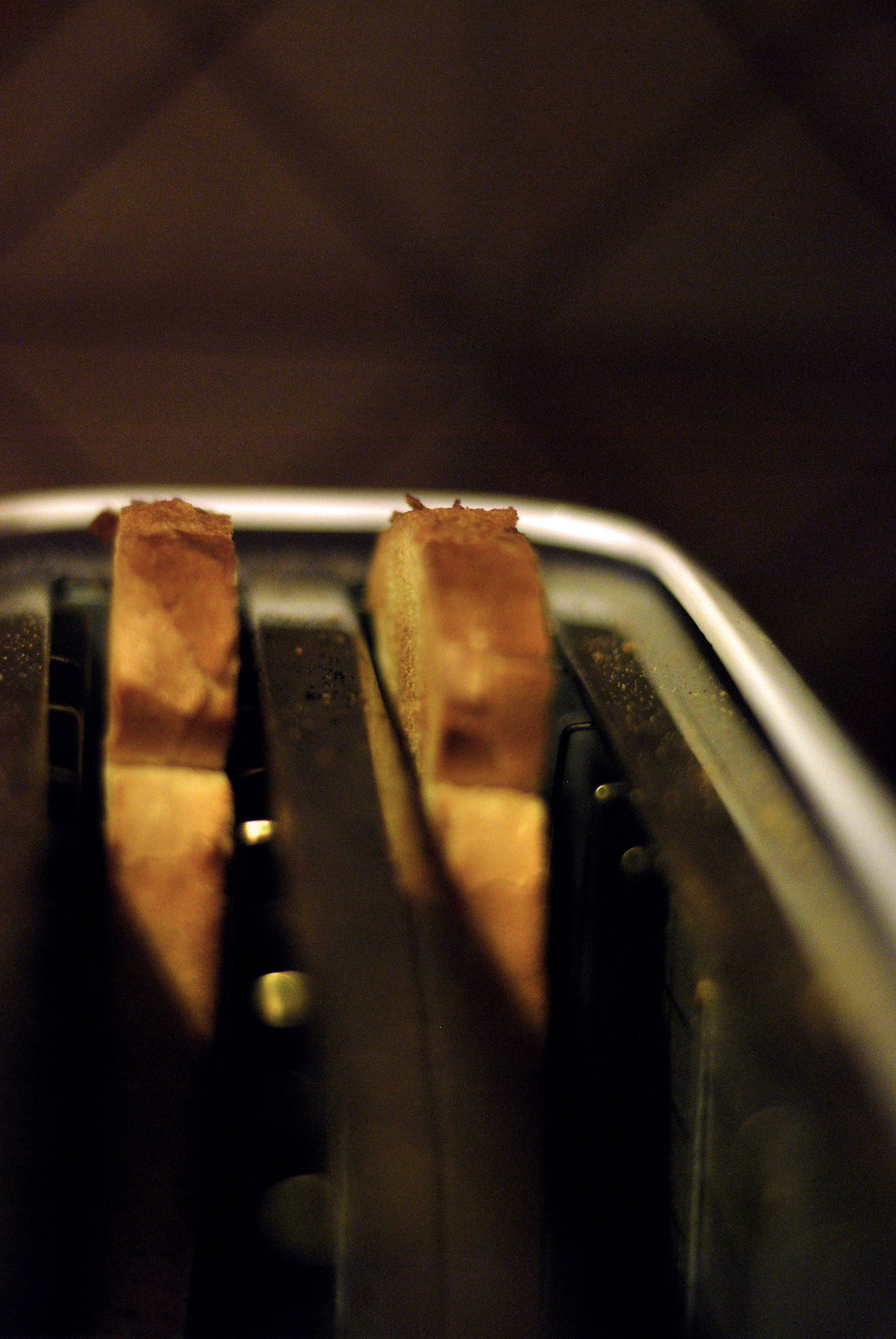The image features a close-up of a stainless steel or chrome toaster with two perfectly toasted slices of white bread. The toast, golden brown with crisp edges, is prominently displayed, partially cropped at the bottom, highlighting its thickness and texture. The toaster slots are wide enough to accommodate thicker bread, adding to the detailed and intentional design of the appliance. The background is dark and slightly blurred, possibly featuring a diamond-patterned wallpaper and a baby gate, creating a cozy and domestic atmosphere. Shadows fall across the bottom part of the toast, accentuating its appetizing appearance. The sleek and shiny toaster contrasts with the darker interior, enhancing the focus on the beautifully toasted bread.